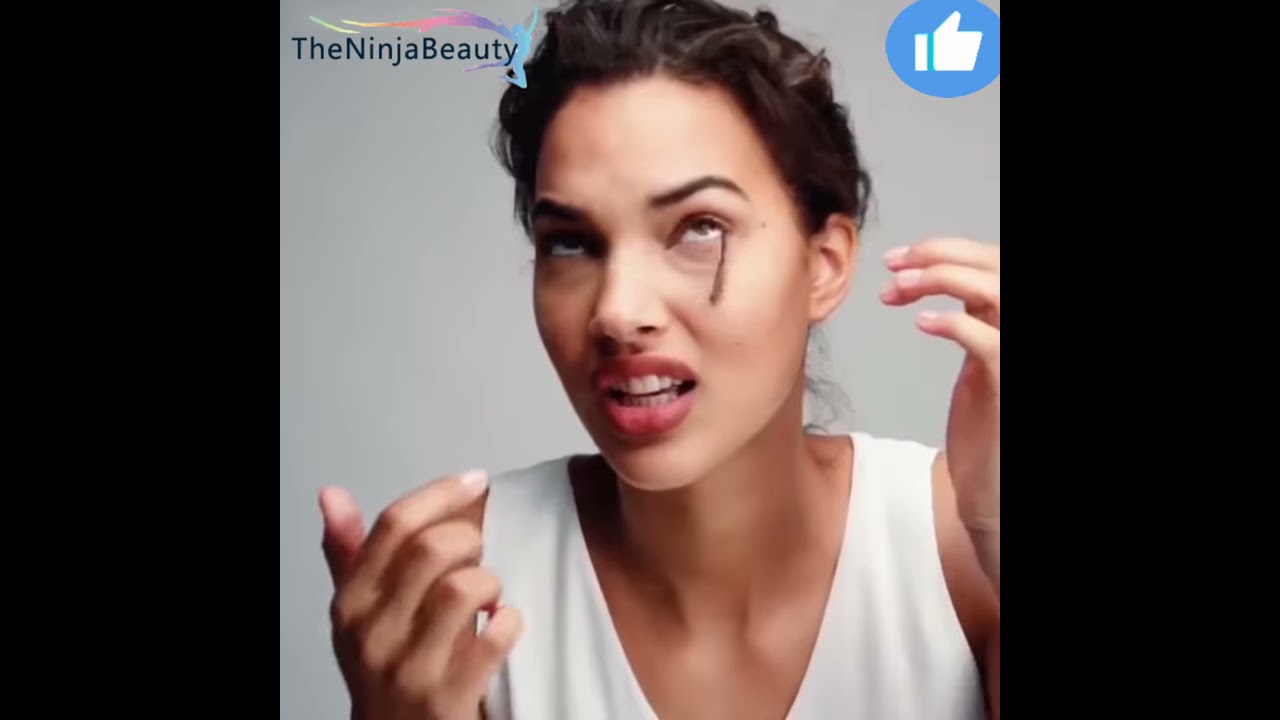The image features a young Caucasian woman with brown hair that is pulled back, creating a wispy appearance at the nape of her neck. She is dressed in a white sleeveless V-neck shirt. Her expression shows a mixture of exasperation and disgust, with her mouth slightly open and teeth visible. Her eyes are directed upwards, and one of her false eyelashes is falling down her left cheek, accompanied by streaks of mascara or eyeliner. Her hands are raised and positioned near her face, suggesting a frantic or surprised motion. The backdrop of the image is a light silver-gray wall, bordered by black strips on both the left and right edges. 

In the upper left-hand corner, the text "The Ninja Beauty" is written in black print, embellished with a colorful ribbon featuring swirls of purple, pink, orange, and yellow, concluding with a blue image of a dancing figurine. The right corner holds a blue circle with a white thumbs-up icon. The overall design suggests a promotional or influencer-themed picture, possibly related to makeup or beauty products.